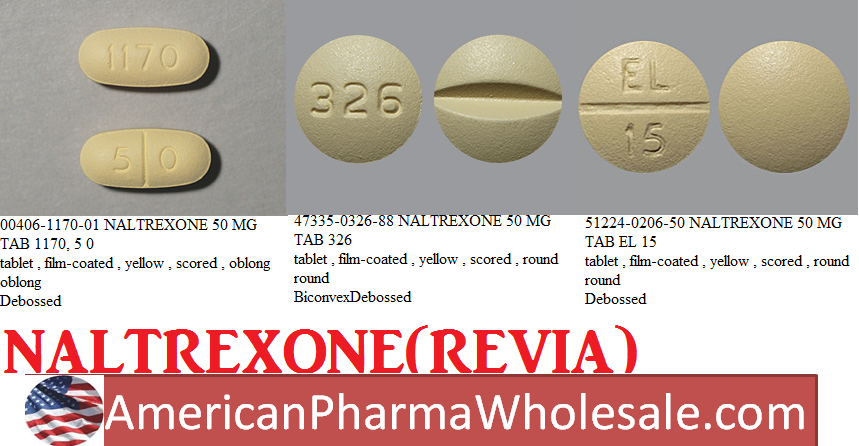This online advertisement for AmericanPharmaWholesale.com features a prominently displayed American flag logo next to the website address at the bottom of the page. The focus of the advertisement is on the drug Naltrexone, also known by the brand name Revia. The name is clearly spelled out as "Naltrexone (Revia)" to indicate the dual identification, though it is unclear which is the brand name and which is the generic.

The advertisement showcases three different variants of Naltrexone 50mg tablets, each accompanied by an image and a brief description. The first variant is labeled simply as Naltrexone 50mg with the brand name DeBost. The second one is described as Naltrexone 50mg Biconvex DeBost, highlighting its tablet shape. The third variant is also listed as DeBost without additional description.

AmericanPharmaWholesale.com is a platform for purchasing wholesale pharmaceuticals, and this specific page focuses on Naltrexone tablets, detailing their availability and presentation.